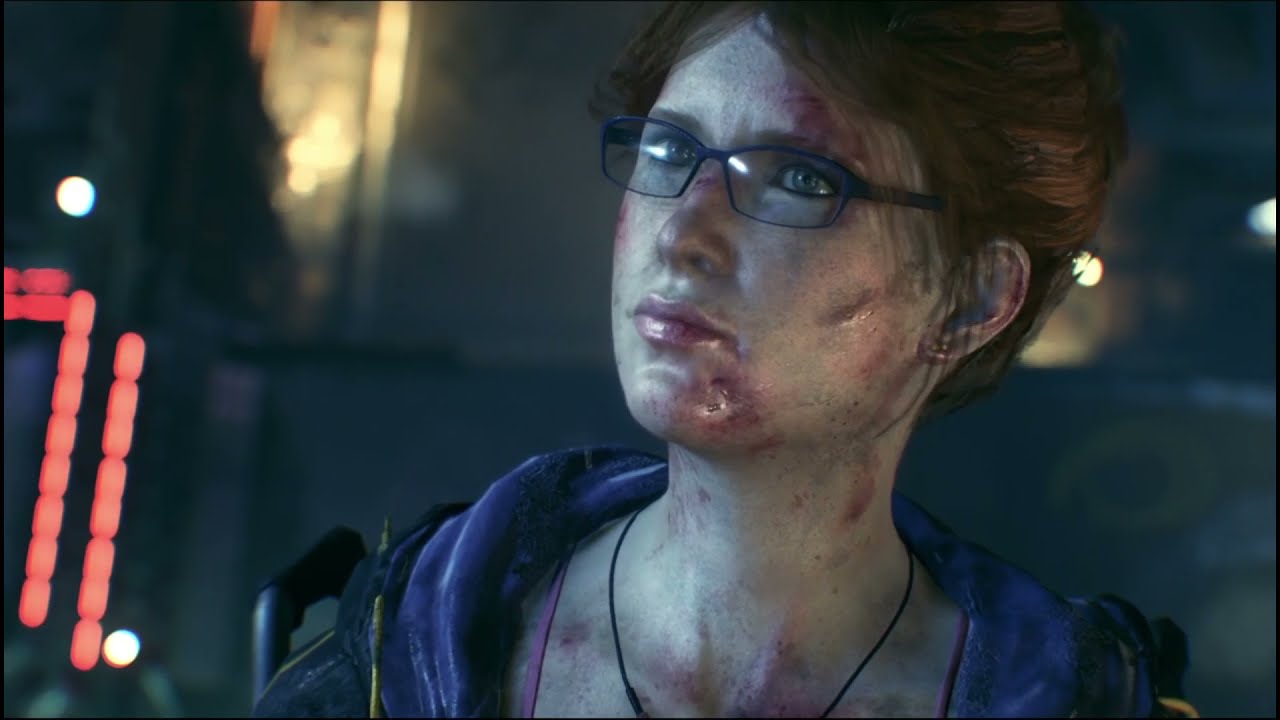This vividly detailed 3D rendered image depicts a close-up of a badly beaten and bruised white woman with brown hair tied up in a bun, wearing glasses. She has conspicuous cuts on her face, blood trickling from her chin and lips, and visible scuff marks as well as dirt on her face, neck, and chest. Her attire consists of a blue hoodie, and a necklace can be seen encircling her neck, though the pendant is not visible as the image cuts off around her chest. Intense light reflections are noticeable on her face and glasses, emphasizing her injuries. She gazes to her right (the viewer’s left). In the indistinct background, which appears to be an urban, outdoor setting, there is a concrete building, a tree, and peculiar red lights or possibly a red electrical sign to the left. A partially visible backpack or suitcase is discernible behind her. The overall scene suggests she has endured a traumatic event, rendering her appearance both gritty and immersive within its digital environment.